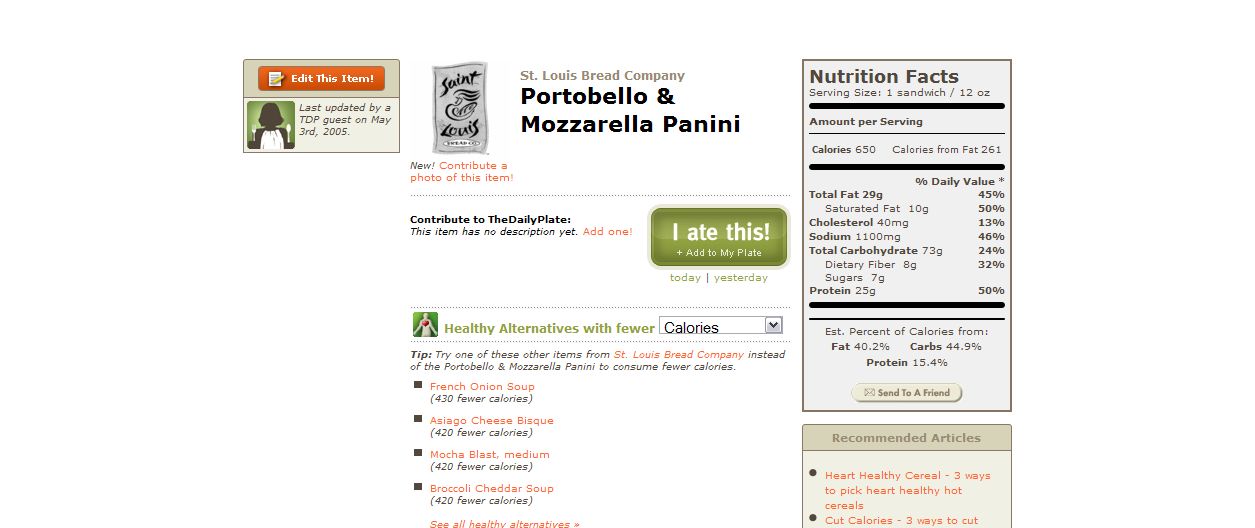**Descriptive Caption:**

The image is a detailed screenshot of a website. On the left side, a small rectangle contains a bright orange rectangle with an icon of a paper and pencil on the left side next to white text that reads "Edit This Item!" Below this, there is a silhouette of a person holding a white fork and spoon, wearing a white bib. Adjacent to this, the text reads "Last updated by a TDP guest on May 3, 2005."

Centrally, the words "St. Louis Bread Company, Portobello, and Mozzarella Panini" are prominently displayed. To the left of this is a gray vertical rectangle with the words "St. Louis" and an image depicting a person with long hair holding a piece of bread. Beneath this, black text reads "new!" and below, in orange, "contribute a photo of this item." Further down, it states in black, "Contribute to the daily plate." This item currently lacks a description, as expressed in the text "This item has no description yet." Orange text invites the user to "Add one."

On the right side, a green rectangle features the words "I eat this!" and "Add to my plate" in white. Below, green text says "Today" followed by a black vertically oriented orange line, then "Yesterday" in green. Below this is a section titled "Healthy Alternatives" with the words "Fewer" in green and "Calories" in red, listed within a drop-down menu.

The following section suggests healthier alternatives available at St. Louis Bread Company to the Portobello Mozzarella Panini to reduce calorie intake. Bulleted items include:
- French Onion Soup (430 fewer calories)
- Asiago Cheese Bisque (420 fewer calories)
- Mocha Blast, Medium (420 fewer calories)
- Broccoli Cheddar Soup (420 fewer calories)

In red text at the bottom, it says "See all healthy alternatives" with two arrowheads pointing to the right.

On the far right, a rectangle details the "Nutrition Facts" in black. It includes:
- Serving Size: 1 sandwich (12 ounces)
- Amount Per Serving
- Calories: 650 (with Calories from Fat: 261)
- Total Fat: 29 grams, 45%
- Saturated Fat: 10 grams, 50%
- Cholesterol: 40 milligrams, 13%
- Sodium: 1,100 milligrams, 46%
- Total Carbohydrate: 73 grams, 24%
- Dietary Fiber: 8 grams, 32%
- Sugars: 7 grams
- Protein: 25 grams, 50%
- Estimated Percent of Calories from: Fat 40.2%, Carbs 44.9%, Protein 15.4%

A yellow rounded rectangle labeled "Send to a Friend" appears underneath.

Below this is a rectangular box titled "Recommended Articles" listing:
- "Heart Healthy Cereal"
- "Three Ways to Pick Heart Healthy Hot Cereals"
- "Cut Calories - Three Ways to Cut"